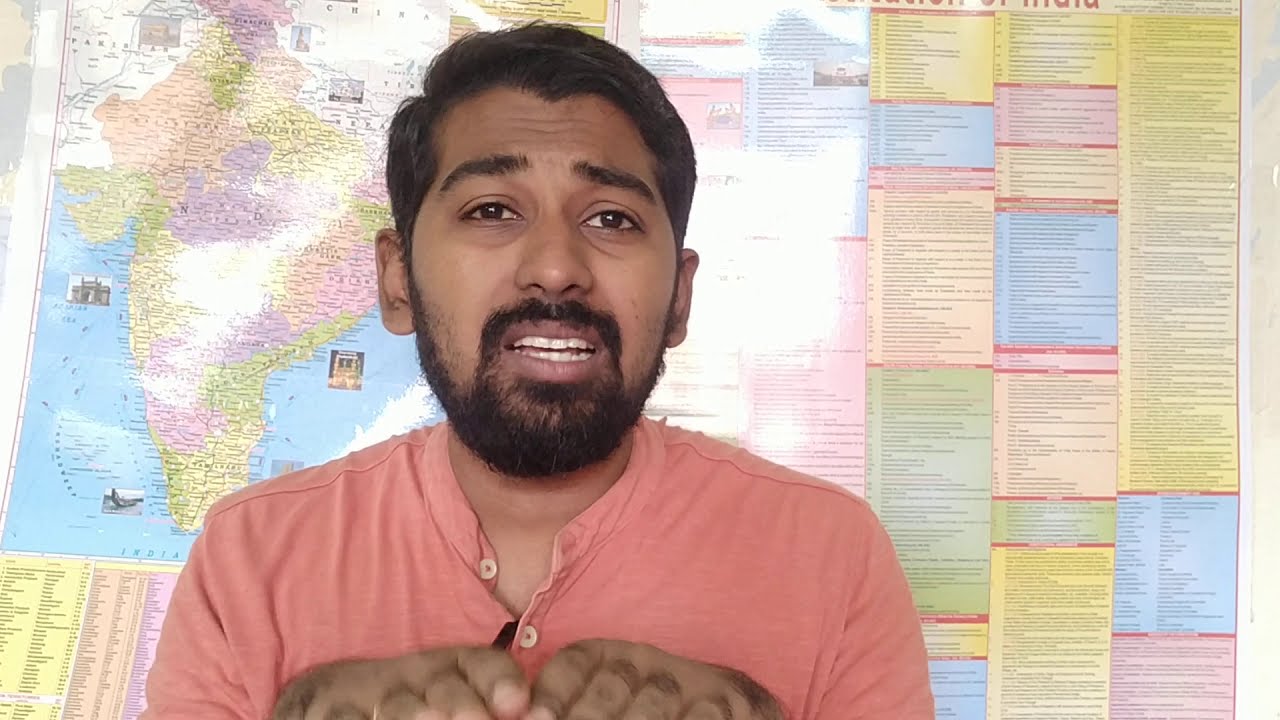In this image, a man is positioned towards the center, slightly off to the left. He is dressed in a light pink or salmon-colored button-down shirt with the top buttons undone. The shirt features a circular collar, and only the upper part of his torso, up to his chest, is visible. His hands, partially in view, are raised in front of him, suggesting a motion of explanation. He has short, dark hair, brown eyes, and a black beard with a matching mustache and goatee. His facial expression is a mix of curiosity and subtle sadness, with raised eyebrows and slightly open mouth, as though he is in mid-conversation or about to ask a question.

The background prominently features a large map, identified as a detailed map of India. The map occupies the left side of the image, while the right side and lower left corner have numerous color-coded text boxes and columns, likely providing extensive information related to the map. The text and map suggest an educational setting, potentially a classroom or lecture room. The man’s engaged demeanor and the intricate map with its detailed legend indicate he might be explaining or discussing something related to the geographical and cultural aspects of India.